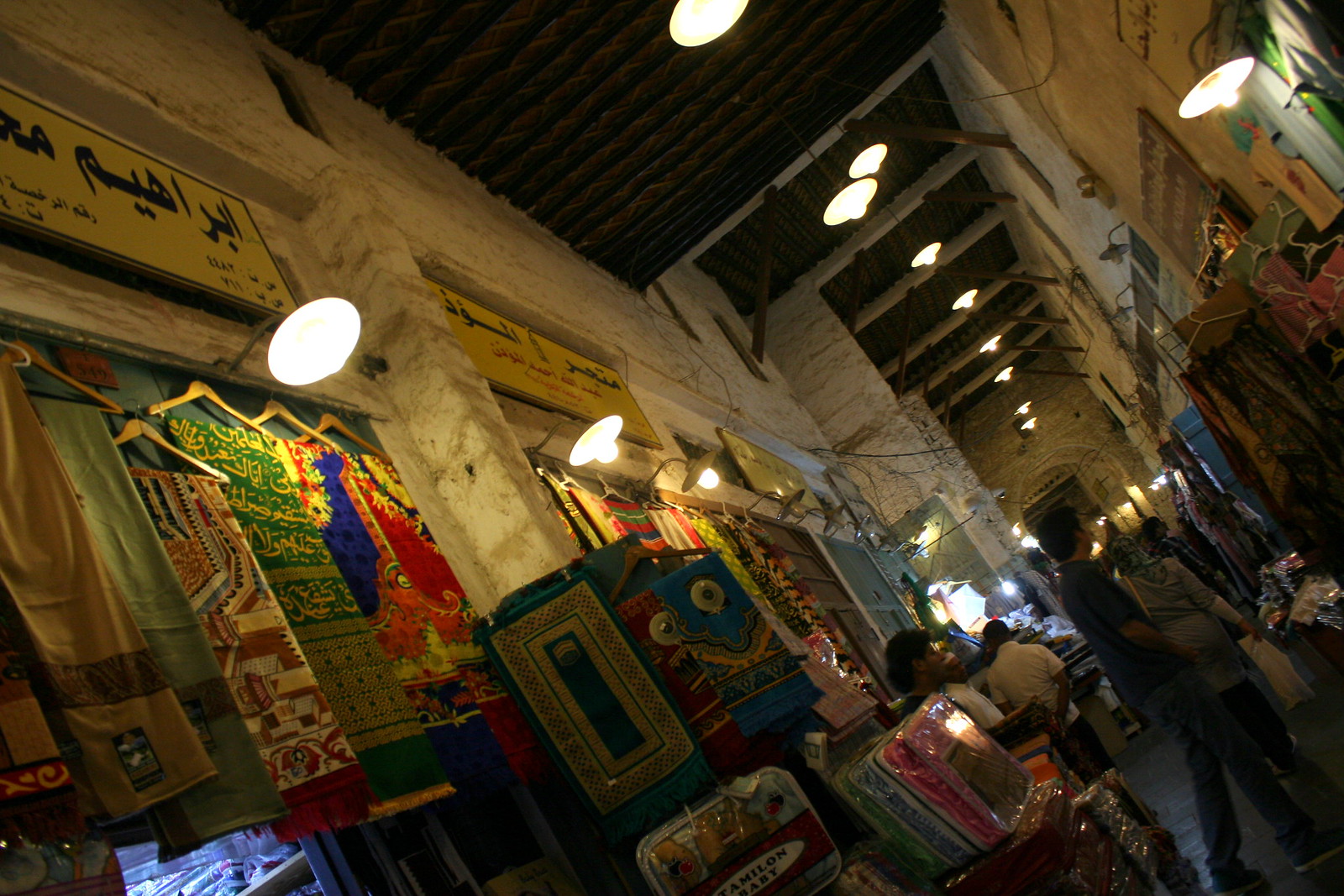The photograph captures a bustling interior corridor of a marketplace building, showcasing a vibrant array of cultural elements. The image is taken at a diagonal angle, adding a dynamic perspective to a scene filled with activity. Overhead, various signs written in a non-English language provide visual clues to the diverse offerings within the marketplace. The corridor is adorned with hanging lights that illuminate the array of goods displayed prominently on both walls.

On the left and right sides, there are numerous items for sale, including an assortment of colorful clothing and textiles hung from racks and displayed on hangers. The scene is populated with several individuals walking through the corridor. Notably, a gentleman clad in a white t-shirt strides along, while a woman, her head modestly covered with a scarf, carries a bag, suggesting she might be shopping or exploring the marketplace. The overall ambiance exudes a lively and authentic marketplace experience, rich with cultural nuance and local flavor.